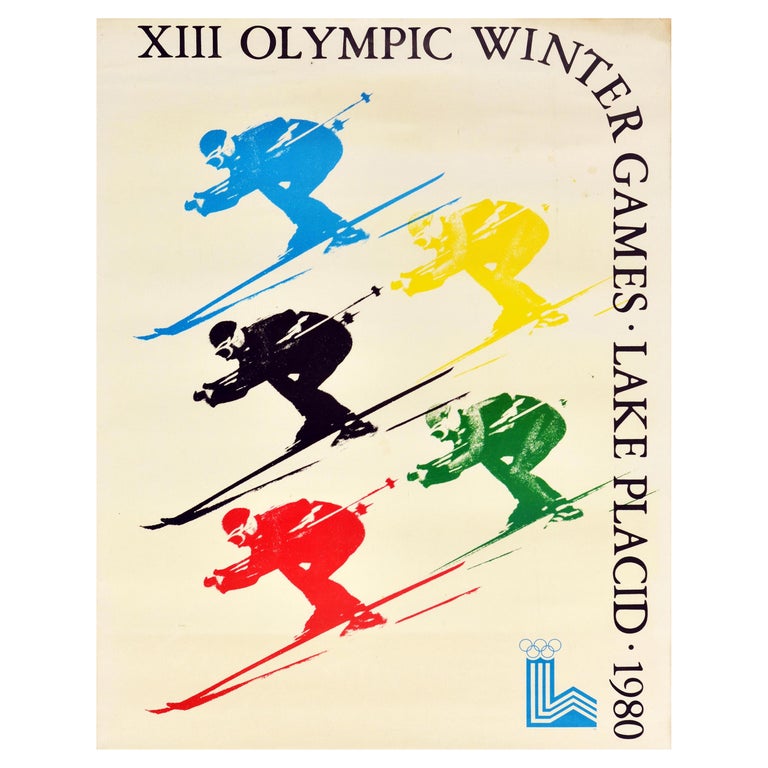This is a detailed poster for the XIII Olympic Winter Games held in Lake Placid, 1980. The background is a soft beige. The text starts at the top, with "XIII Olympic Winter" written across, then moves to the right edge with "Games.LakePlacid.1980" wrapping downwards. The central graphic features five identical skiers in a dynamic, downhill skiing pose. Each skier is in a different bold color: blue at the top, followed by black, yellow, red, and green. In the bottom right corner, the Olympic emblem is prominently displayed, featuring the iconic rings atop three blue lines resembling a podium. The clean and repetitive imagery of the skiers, along with the stylistic text layout, creates a striking and cohesive visual representation of the 1980 Winter Olympics.